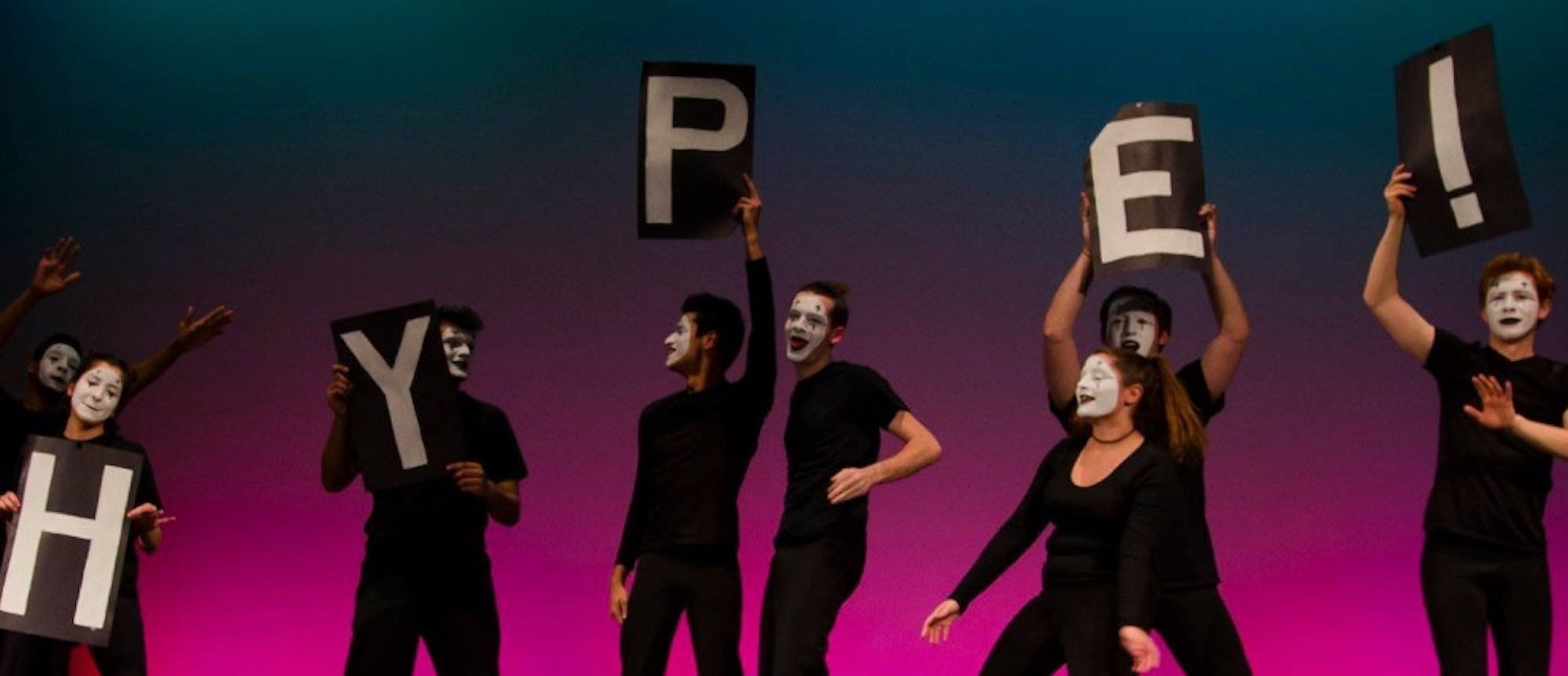The rectangular photograph captures the dynamic scene of an indoor theatrical performance, likely taking place on a stage. The background is illuminated by a striking gradient, transitioning from navy blue at the top to a vivid purple hue at the floor level. The stage features eight young performers, both male and female, dressed uniformly in solid black attire, including pants and varying styles of shirts, predominantly short-sleeved. Their faces are strikingly painted white with black accents around their eyes and lips, mimicking the makeup of mimes. Each performer is holding a black sign with a bold white letter printed on it. From left to right, the letters spell out "HYPE" followed by an exclamation mark. The ensemble seems to be engaged in expressive movements or a dance, contributing to the lively atmosphere. The backdrop enhances the visual impact with its magenta-to-dark cyan gradient, adding depth and vibrancy to the overall composition.